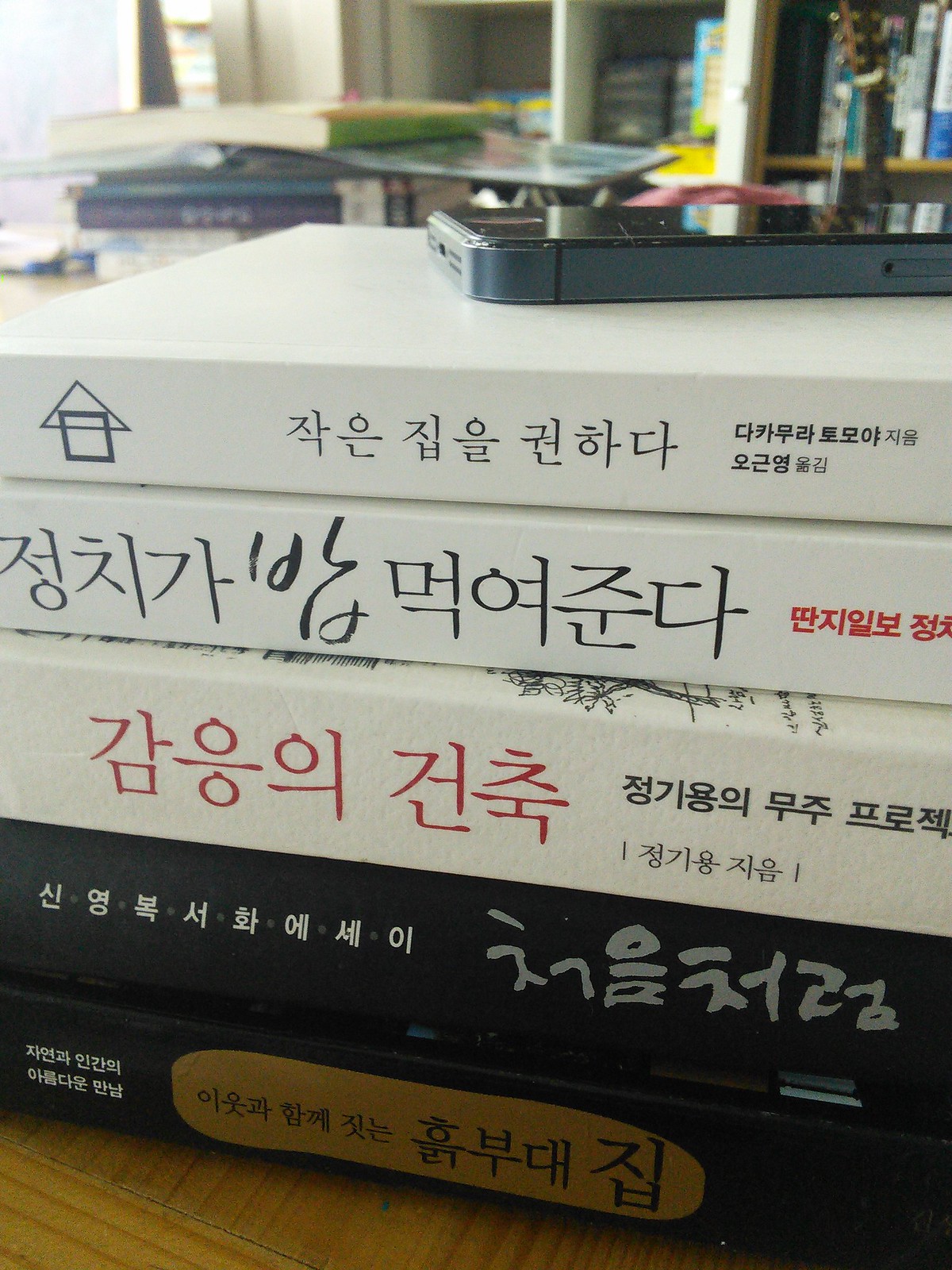The image captures a brightly lit indoor setting, possibly an office or home workspace. Central to the photograph is a stack of five books on a light-colored wooden table, with their spines featuring what appears to be Chinese or Japanese characters. The top three books are predominantly white with black and red lettering, while the bottom two books are black, with the lowest one having a gold, oval-shaped banded area on its spine. Positioned at an angle atop the stack is a black cell phone. In the background, there are bookshelves filled with vertically and horizontally arranged books, interspersed with papers and the neck of a guitar. The room is well-lit, with natural light flooding in possibly from a window in the upper left corner.